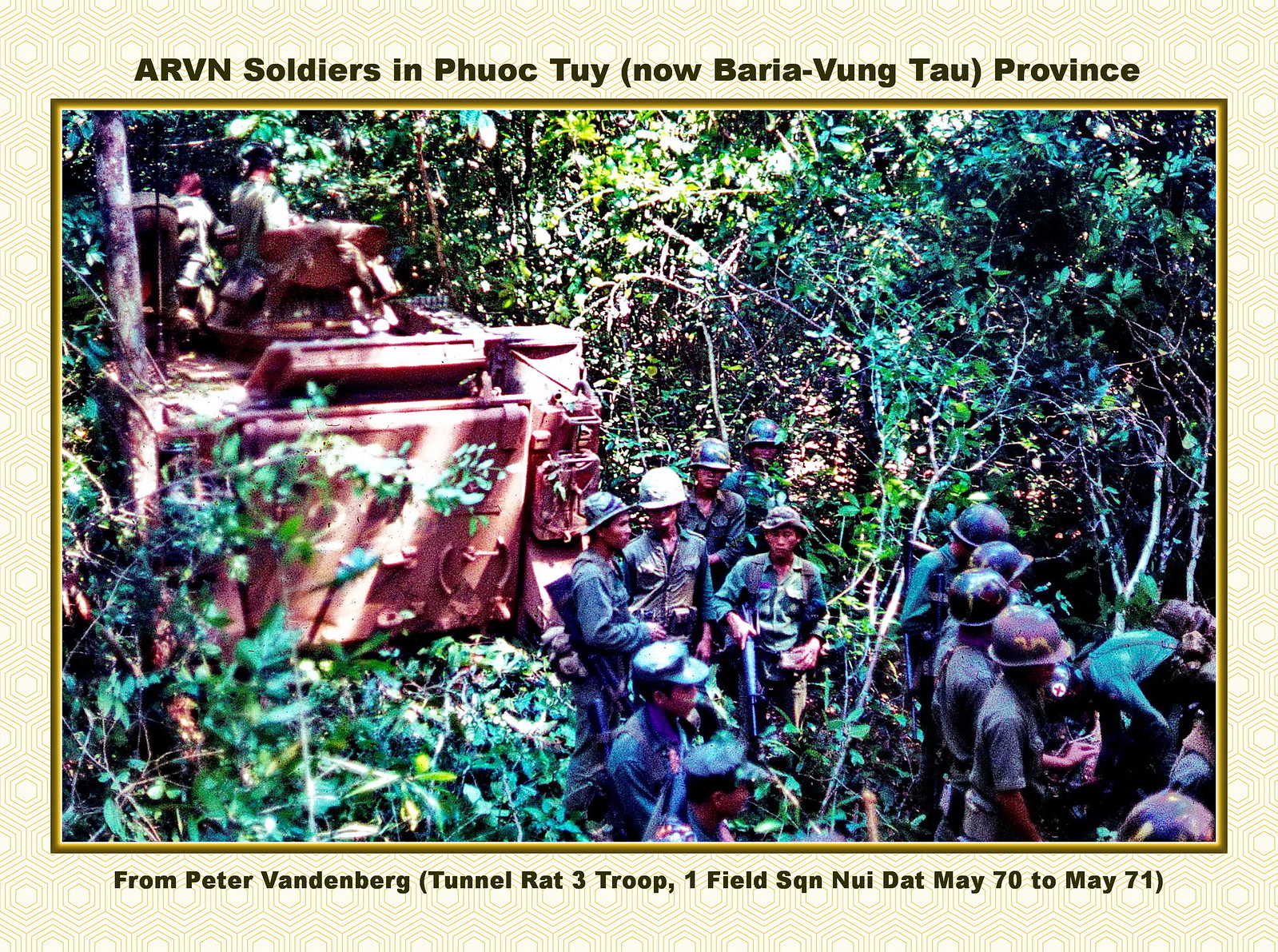Caption: 

An intriguing vintage postcard captures a group of soldiers navigating through dense jungle terrain, likely in Vietnam, given the military context. The scene is reminiscent of the Vietnam War era, specifically around May 1970-1971. The soldiers are equipped with substantial, potentially heavy-duty military gear, essential for maneuvering through challenging woodland environments. The backdrop features intricate patterns and a distinct golden tone, enhancing the historical richness of the image. This evocative photo offers a glimpse into the past, highlighting the arduous journey of troops during a significant period in history.